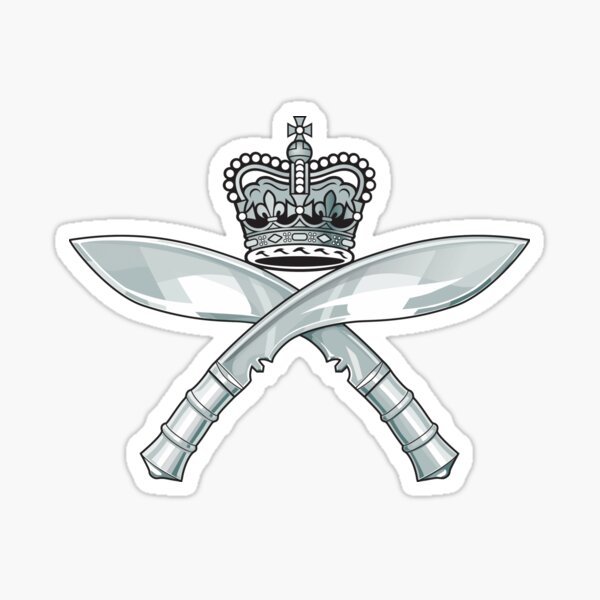This detailed grayscale illustration, resembling cut-out art or a sticker, features a prominent and ornate emblem. At its center, two kukri-like blades are crossed in an X formation, their silvery gray, teardrop-shaped ends shining with a metallic sheen. Above these intersecting swords stands a regal king's crown. This crown boasts intricate details: a base ring adorned with circles that may represent beads or gems, an arced crest rising to a ball, and an iron cross perched atop the ball. The entire image, bordered in black and white and set against a stark white background, suggests a dignified insignia or brooch, suitable for adorning a dress or suit. The meticulous pencil-like shading and grayscale tones lend the piece a classic, ornamental quality.